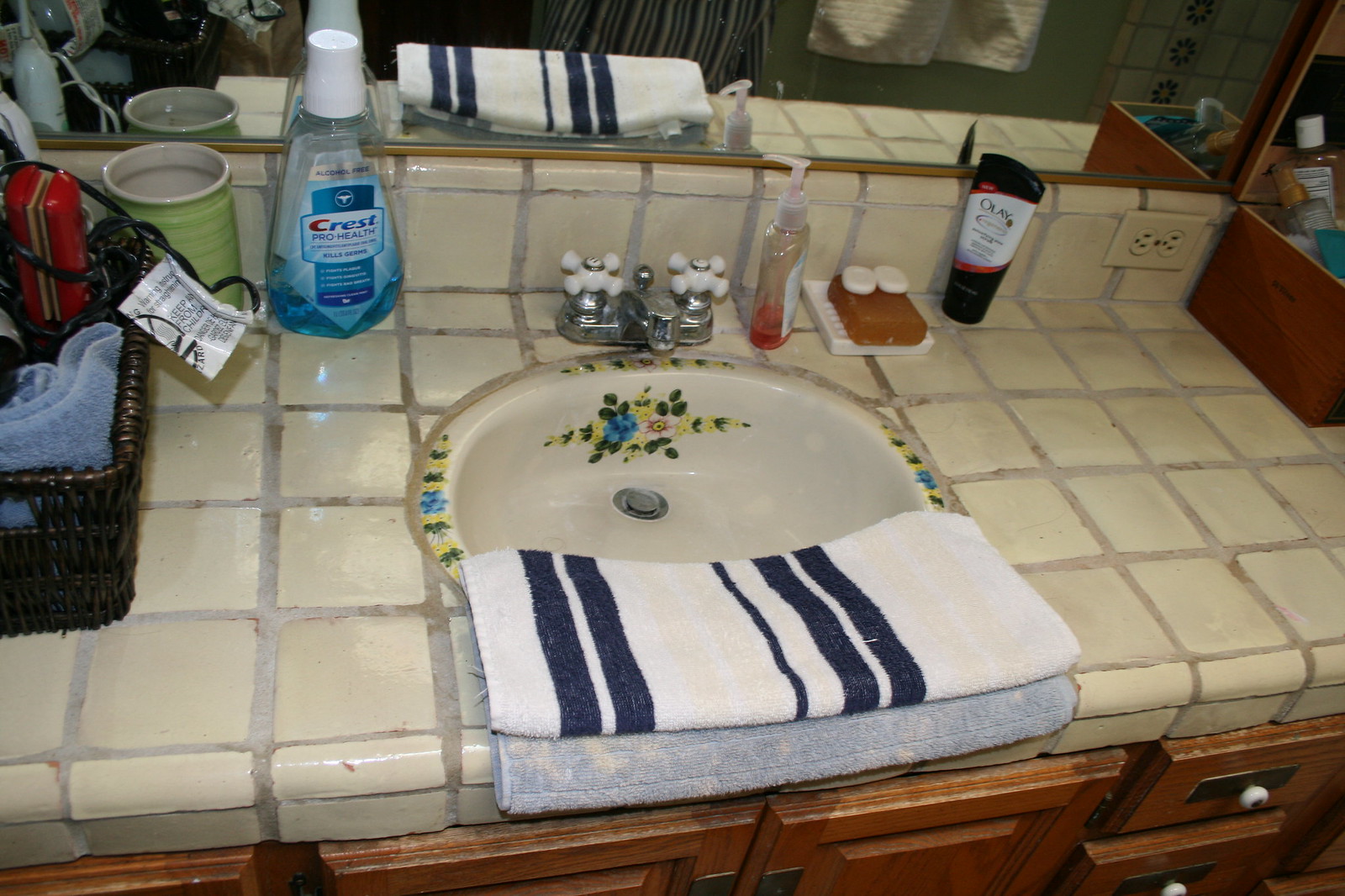This image showcases a bathroom sink situated on a white tile countertop. To the left of the sink, a brown wicker basket contains a blue washcloth or towel, alongside a red flat iron with a black cord. Positioned on the sink is a green ceramic mug, likely a candle holder. Nearby, a bottle of Crest Pro Health mouth rinse stands next to a hand soap dispenser with a small amount of orange liquid soap remaining inside. A white soap dish lies on the countertop, containing an orangish-brown bar of soap, potentially Neutrogena, topped with two small white soap bars. A bottle of Olay moisturizer or lotion is also present. The sink itself features a floral motif with yellow, green, blue, and pink flower designs. Draped in front of the sink are two towels—a white towel with blue stripes folded on top of a light blue towel that shows some staining.